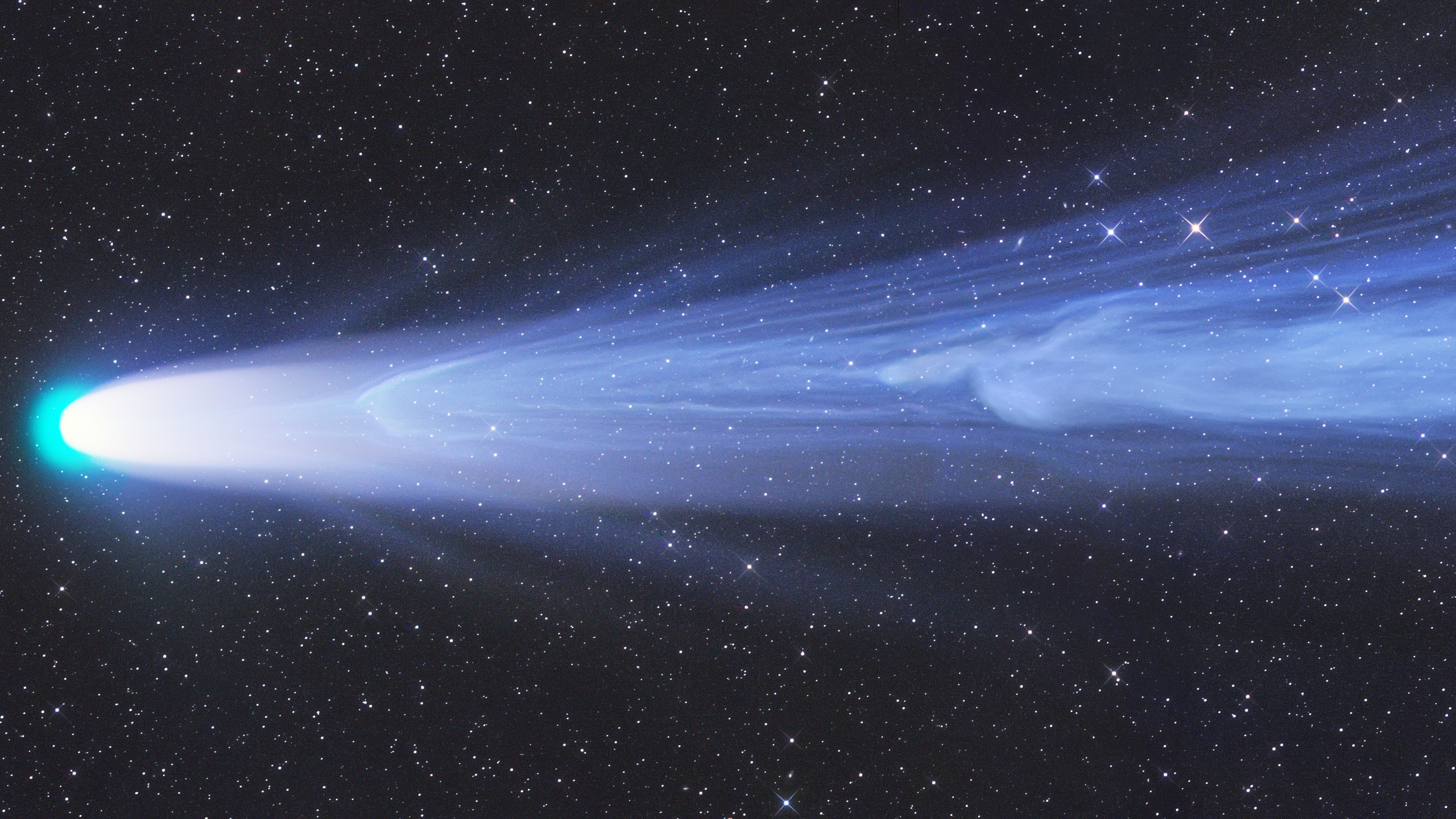In this image, a brilliant white comet, often referred to as the "white hawk comet," traverses the vastness of space from right to left against a pitch-black background sprinkled with a multitude of stars. The comet's head is notably dense and has a sky-blue hue at its tip, which almost looks like a covering over the end of the luminous ray trailing behind it. This ray of light fans out into what appears to be a long, somewhat translucent tail, which remains densely white near the head before fading and then becoming denser again at its end. The tail stretches across the image, contrasting vividly with the backdrop. Alongside the comet, brighter and more pronounced stars dot the path, accentuating the comet's journey. The entire scene captures the comet's dynamic movement, with the left part of the image showcasing a mysterious turquoise orb-like shape at the head, surrounded by a fluffier, smoke-like texture, adding a surreal touch to the celestial spectacle.